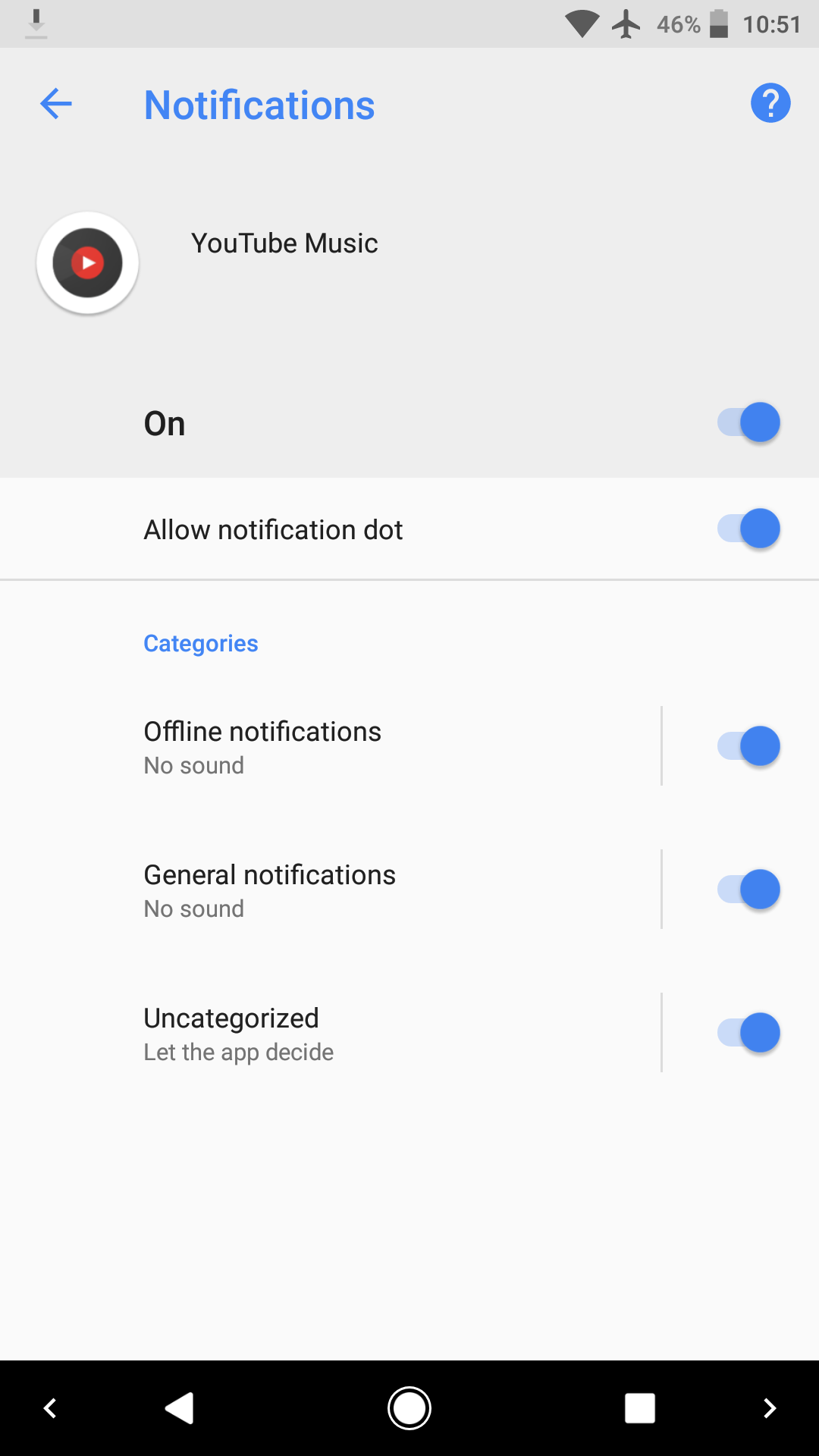Here is a cleaned-up and detailed descriptive caption:

---

This mobile phone screenshot shows the YouTube Music application interface. The top of the display features various icons: the Wi-Fi icon, indicating a Wi-Fi connection despite the phone being in airplane mode, a battery icon showing 46% battery life, and the time displayed as 10:51 AM. To the far left, an underlined microphone icon is visible.

Beneath the top bar, there is a lighter gray box, slightly darker than the top bar, which contains the word "Notifications" in blue, accompanied by an arrow pointing left and a question mark inside a blue circle. Below this section, there is an image representing YouTube Music that includes a record icon with a play symbol (triangle pointing to the right) within the record label, all inside a white circle.

Further down, a series of labels and toggle buttons indicate the notification settings for YouTube Music. The "Allow notifications" switch is toggled on, followed by a faint gray line. The "Categories" section includes the option "Offline notifications," marked as 'no sound' and switched on, separated by another gray line from "General notifications," also labeled 'no sound,' and switched on. Lastly, the "Uncategorized" section with the option "Let the app decide" is switched on.

At the bottom, there are navigation icons displayed on a black background: a less-than sign, a triangle pointing left, a record icon with a play symbol inside two circles, a filled white square, and a greater-than sign, all in white.

---